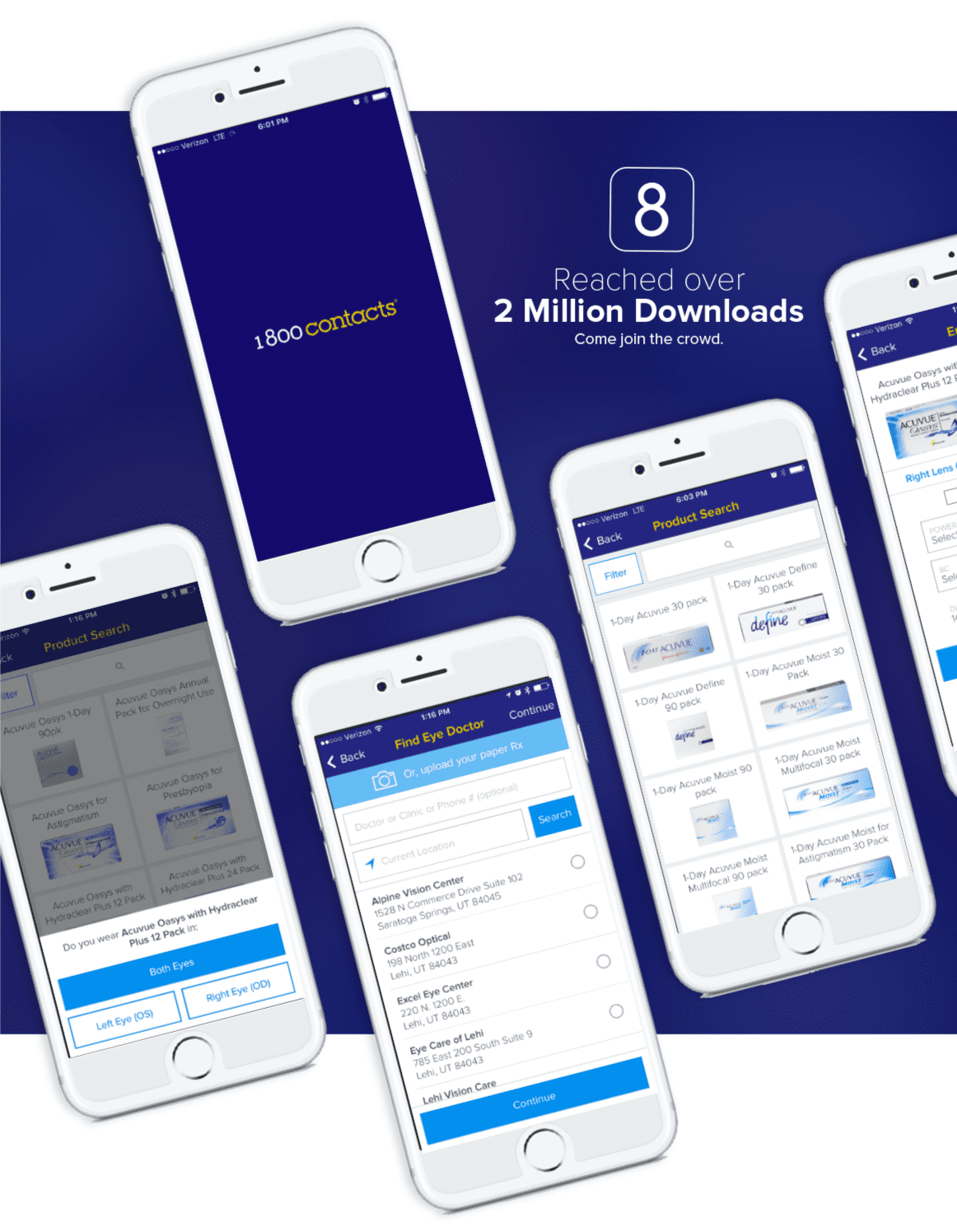This advertisement prominently features a background that transitions from dark blue at the top to white at the bottom. Dominating the upper section, a bold number "8" is outlined and accompanied by the text "reached over 2 million downloads," highlighting a significant achievement. Beneath this, in smaller font, the phrase "come join the crowd" invites viewers to join the large user base. 

The lower section of the advertisement displays several smartphone screens, likely iPhones, each showcasing different content related to the product or service being advertised. One of the phones prominently features a blue background with the text "1-800 Contacts," likely indicating a phone number. These phones are arranged in such a way that some appear against the dark blue background while others extend into the white section, creating a visually engaging and seamless transition across the ad.